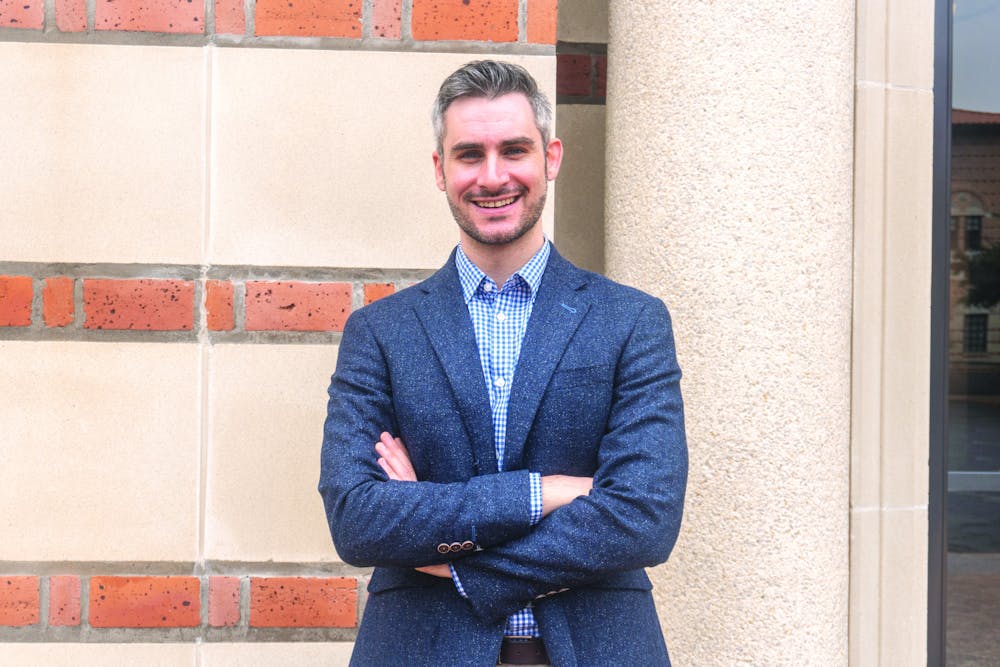In this real-life photograph, a man, dressed in a dark blue suit adorned with small white specks giving it a fancy appearance, is the focal point. Underneath his suit, he wears a blue and white plaid button-up shirt with a collar. The man's arms are crossed, and the image is cropped at around his waist. He stands facing the camera, smiling warmly. He is a white man with a slightly reddish complexion, possibly from embarrassment or natural skin tone. His hair is short, grey, and interspersed with white tufts. His teeth are visible as he smiles.

The background showcases part of a building. To the left of the man, beige sections of the building are interrupted by three singular rows of bricks. On the right side of the frame, a cylindrical pillar can be seen, positioned adjacent to either a glass window or the entryway of the building, featuring dark-tinted glass.